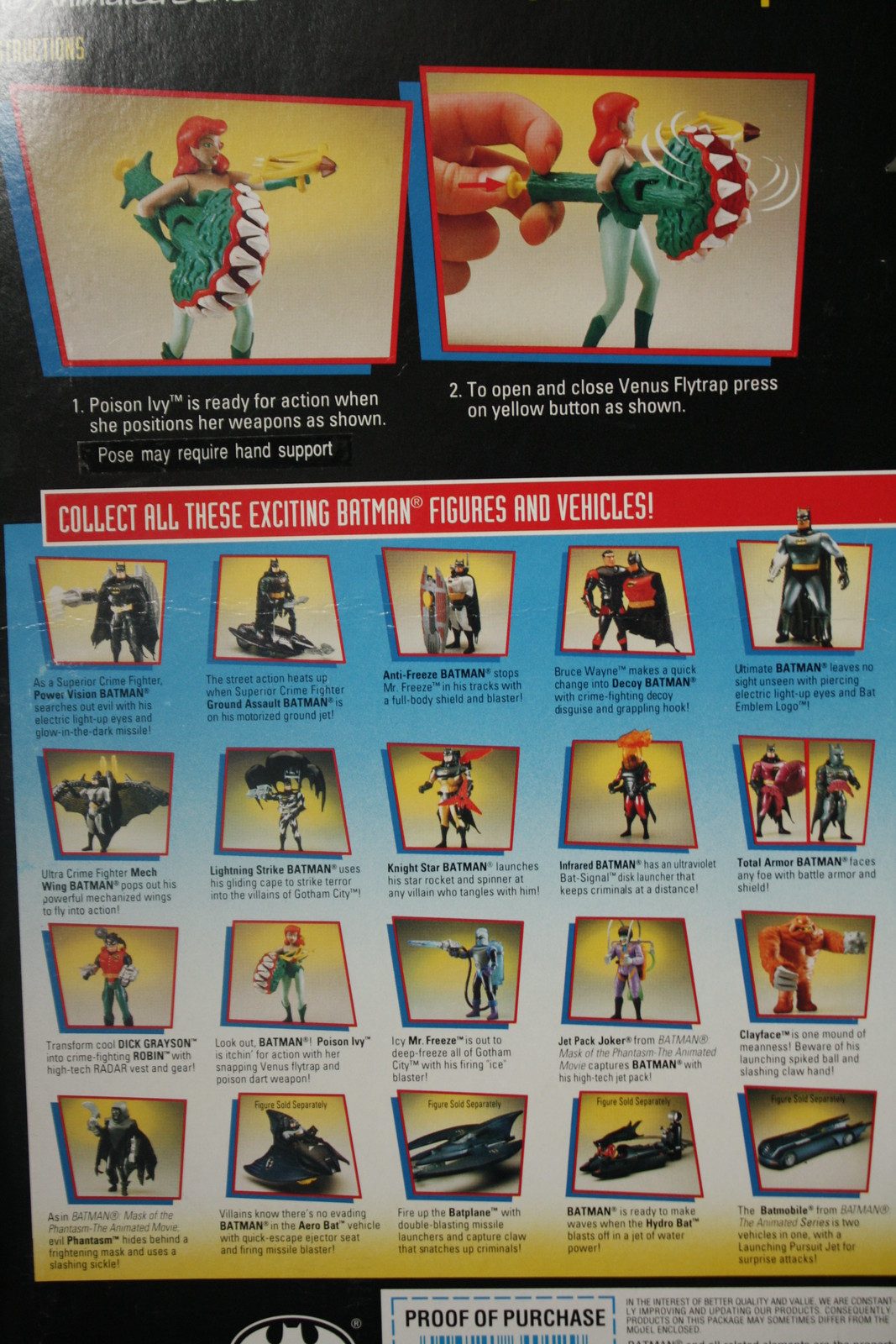The image is a detailed advertisement showcasing a Poison Ivy action figure from the Batman series. At the top, there are two images of the red-haired female figure dressed in green, showing her in different poses holding weapons. In the first image, it states, "Poison Ivy is ready for action when she positions her weapons as shown." The second image depicts Poison Ivy with the same weapons and a human hand pressing a yellow button on a Venus flytrap accessory, with the caption, "To open and close Venus flytrap, press on yellow button as shown." Below these images, there is a section encouraging collectors to "Collect all these exciting Batman figures and vehicles," featuring an array of approximately 15 to 20 different Batman action figures and vehicles, alongside descriptions and a partial view of the UPC proof of purchase code. The Batman logo is also prominently displayed at the bottom.